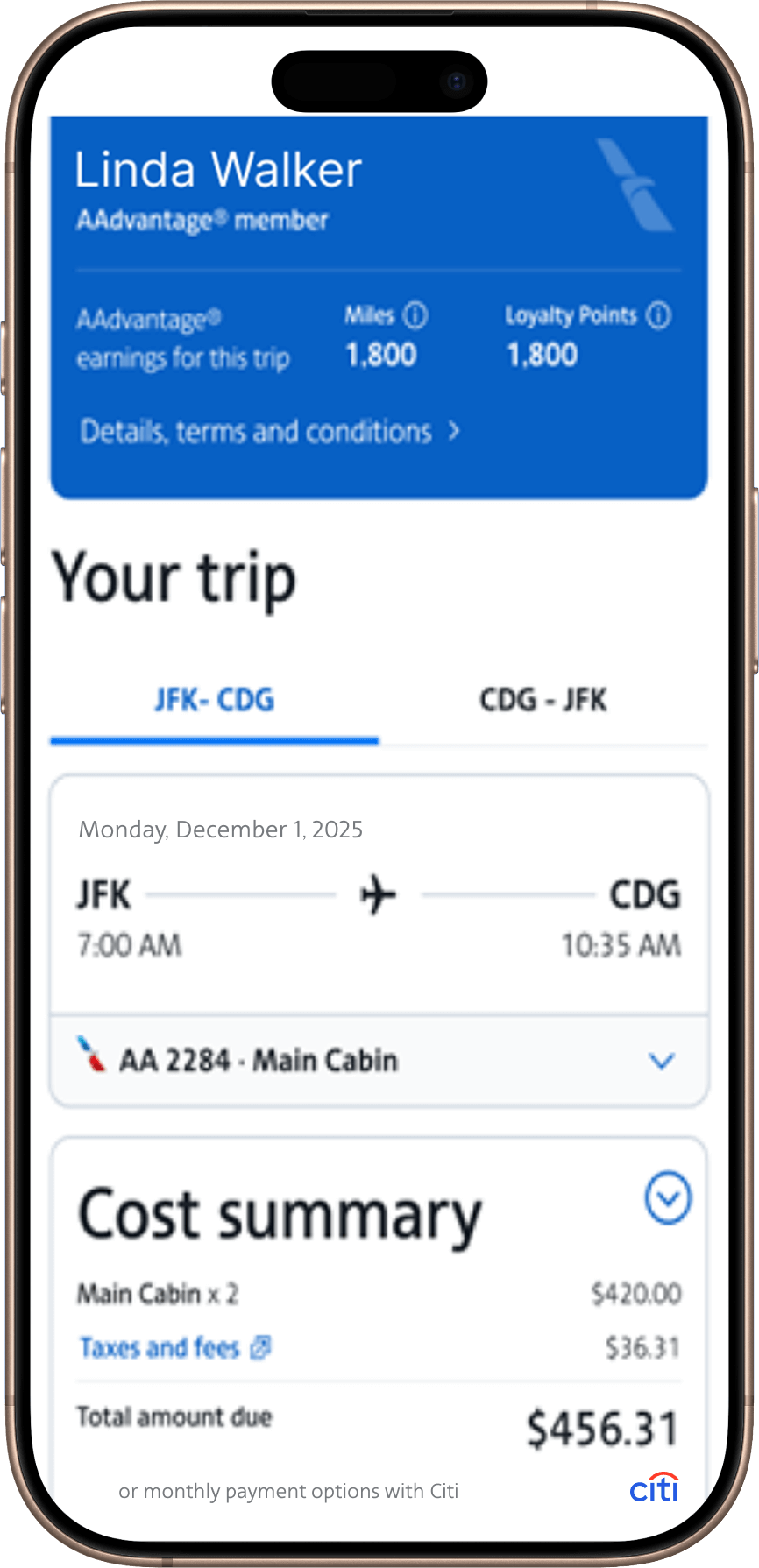The vertically rectangular image showcases a close-up view of a cell phone displaying a detailed travel itinerary for an upcoming flight. The cell phone’s side buttons are visible on both the left and right edges of the device. 

The screen background is primarily white, with essential status icons at the very top: in the top-left corner, the time is displayed as '9:41' in black, while the top-right corner shows signal, Wi-Fi, and battery icons.
 
Below these icons, the screen displays 'American Airlines' in a prominent font. Adjacent to this, on the right side, there is a light blue button labeled 'Lynda Walker'. Beneath this section are interactive options: 'Review and Pay' and 'New Search', aligned to the left. 

Further down, the trip details are presented: travelling from JFK to CDG on Friday, December 1st, 2023, with a 'Details' option highlighted in blue nearby.

Following these details, the 'Your Trip Total' section shows the amount '$456.31', specifying that this total includes all taxes and carrier-imposed fees. 

Directly beneath, there's a 'Cost Details' section, accompanied by a drop-down arrow for expansion. 

At the bottom of the screen, the 'AA Advantage Earnings for This Trip' offers a promotional detail—'Earn 55,000 bonus miles, plus get up to $50 statement credit after qualifying purchases with this credit card offer.' There's also a call-to-action button labeled 'Apply Now'.

The overall design is clean, focusing on providing all necessary information in an accessible manner.